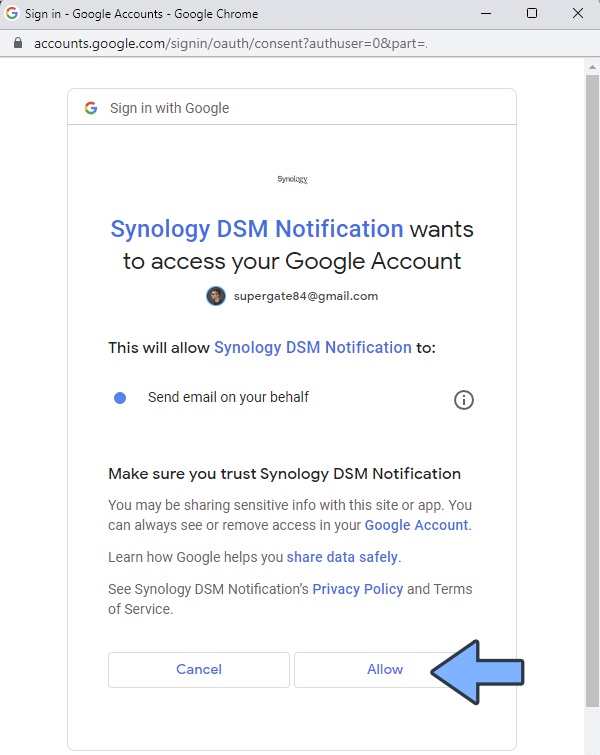The image displays the "Sign in with Google" page in Google Chrome. At the top left, the header reads "Signing in to Google Accounts" and "Google Chrome." Below that, the web address bar shows the URL for the Google Accounts sign-in page: accounts.google.com. Dominating the center is a white box labeled "Sign in with Google" at the top left, accompanied by the Google logo—a multicolored "G."

Beneath this, there is a notification text that says, "Signology DSM notification wants to access your Google Account." In smaller font, the email address "supergate84@gmail.com" is displayed. Following this, there is a disclaimer stating, "This will allow Signology DSM notification to:" with the permission to "Send email on your behalf" listed below. Towards the bottom, a prompt reads, "Make sure you trust Signology DSM notification."

In the lower right-hand corner of the white box, there is an allow button.